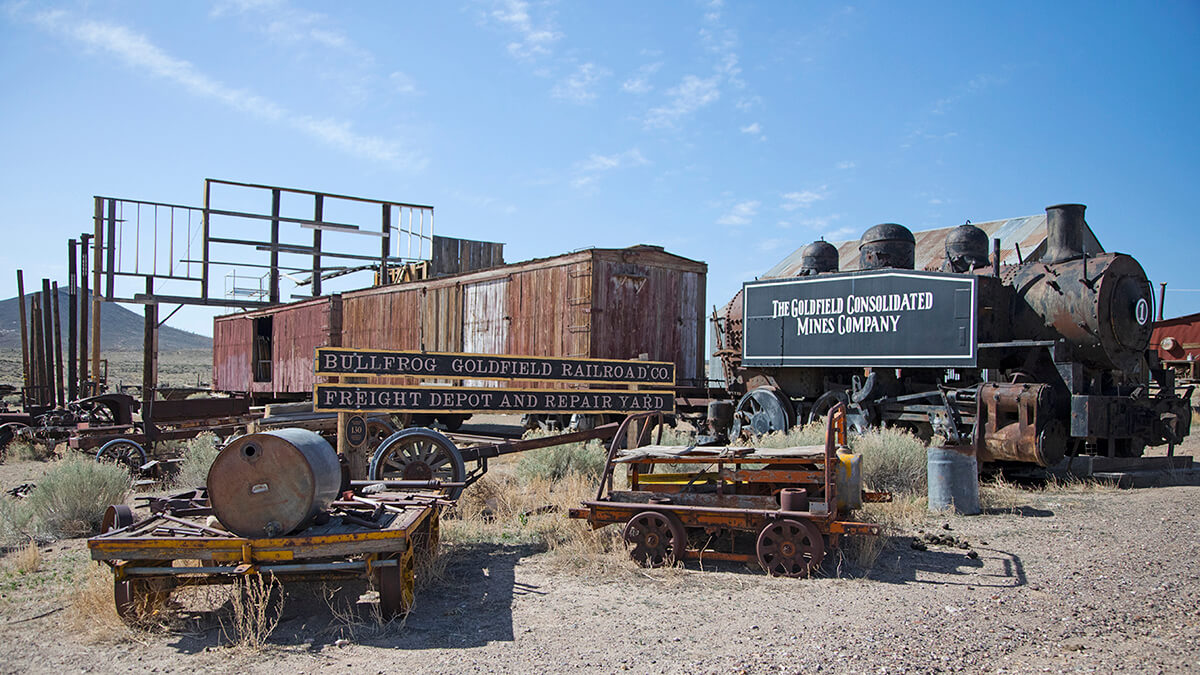The photograph depicts a desolate junkyard situated in the arid landscape of a desert, likely in the western United States. The scene is set under a clear blue sky with minimal vegetation, predominantly brown with sparse green bushes. Central in the image is an old, rusty train engine coupled with a caboose and several faded red train cars, one of which has its door ajar. The rolling stock belongs to the Bullfrog Goldfield Railroad Company, as denoted by an inscription that reads "Goldfield Consolidated Mines Company, Bullfrog Goldfield Railroad Company, Freight Depot and Repair Yard." Surrounding the train are various vintage pieces of machinery, an old wagon, and numerous axles and wheels scattered across the dirt and gravel terrain. In the backdrop, decrepit billboards stand devoid of any readable content, adding to the sense of abandonment. The presence of a barn and distant mountains enhances the historic and forlorn atmosphere of the scene.